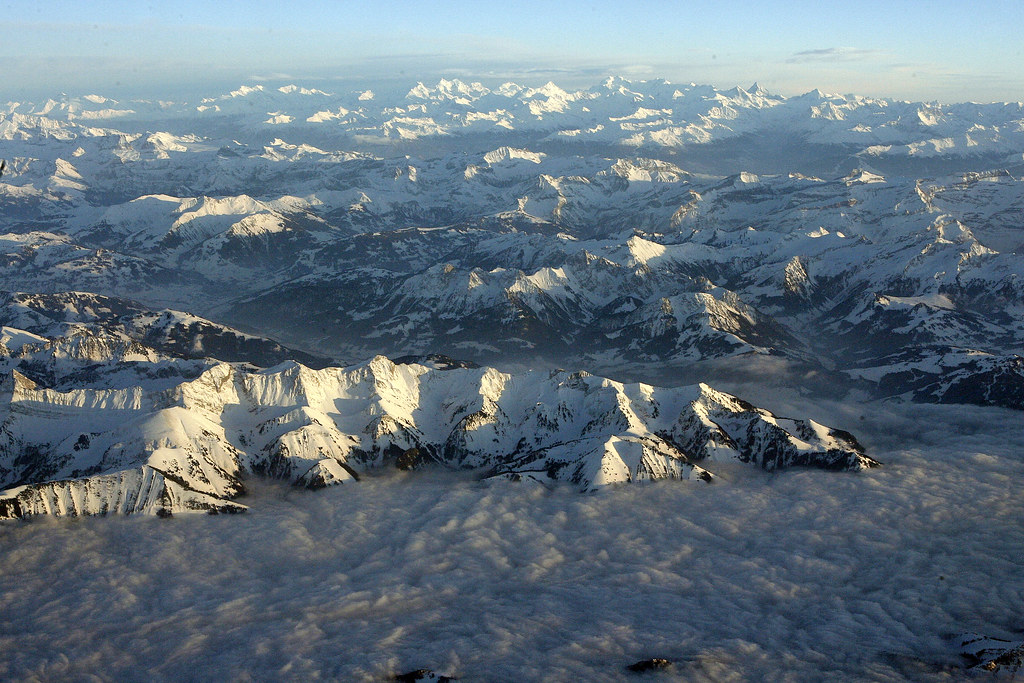The photograph depicts a stunning aerial view of a vast mountainscape dominated by snow-covered peaks, creating a majestic panorama. The scene is painted predominantly in shades of blue and white, with a light blue sky and scattered white clouds overhead. The mountains rise in sharp, snow-capped peaks, their tops glistening under the sunlight, which casts long shadows to the left side of each peak, indicating it is daytime. In the foreground, a dense fog envelopes the nearest mountains, adding to the ethereal quality of the landscape. The image, likely captured from a high altitude or an airplane, hints at a cold region due to the extensive snow cover and the lack of visible vegetation. The mountains extend into the distance, forming a continuous, awe-inspiring chain, with a thin strip of blue sky visible at the horizon. The prominent features of the photograph are the repetitive, snow-covered peaks that create a mesmerizing and serene winter vista.